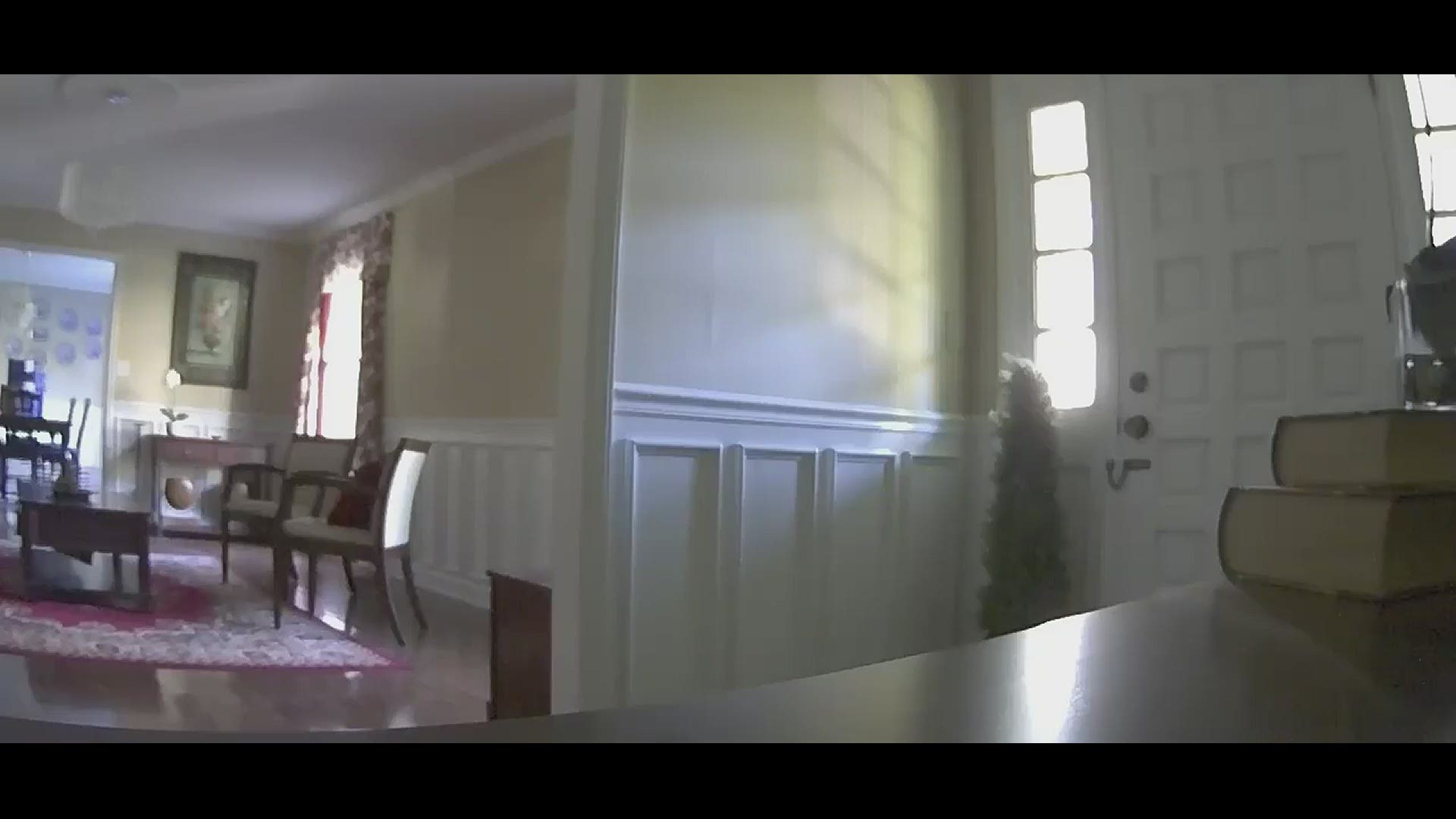This image showcases a well-furnished living and dining area with a cohesive mix of colors and textures. On the right side of the room, a white door with an indented square box detail stands out. The room features two small square windows, each composed of four panes, positioned symmetrically on the left and right. A sidewall partition adorned with white wood paneling runs at the bottom, contrasting with the predominantly white walls. 

In the corner, a small green tree adds a touch of nature to the indoor setting. A sleek silver table on the right holds a stack of two books, enhancing the room's sophisticated atmosphere. The photo itself is framed with black lines at the top and bottom, adding a modern touch.

On the left, red chairs with matching legs and arms provide vibrant seating options. Behind the partition, a brown cabinet peaks out, suggesting additional storage. The living room walls are brown, complemented by white paneling at the bottom. One window is dressed with red and white curtains, adding a pop of color to the space.

The carpet features a purple and white design, and a small square brown table sits in its center. The flooring has a glossy, glass-like brown finish that adds elegance to the room. Overhead, a white light fixture illuminates the space, hanging from the white ceiling. To the right, a green picture decorates the wall above a small brown side table, completing the room's well-thought-out decor.